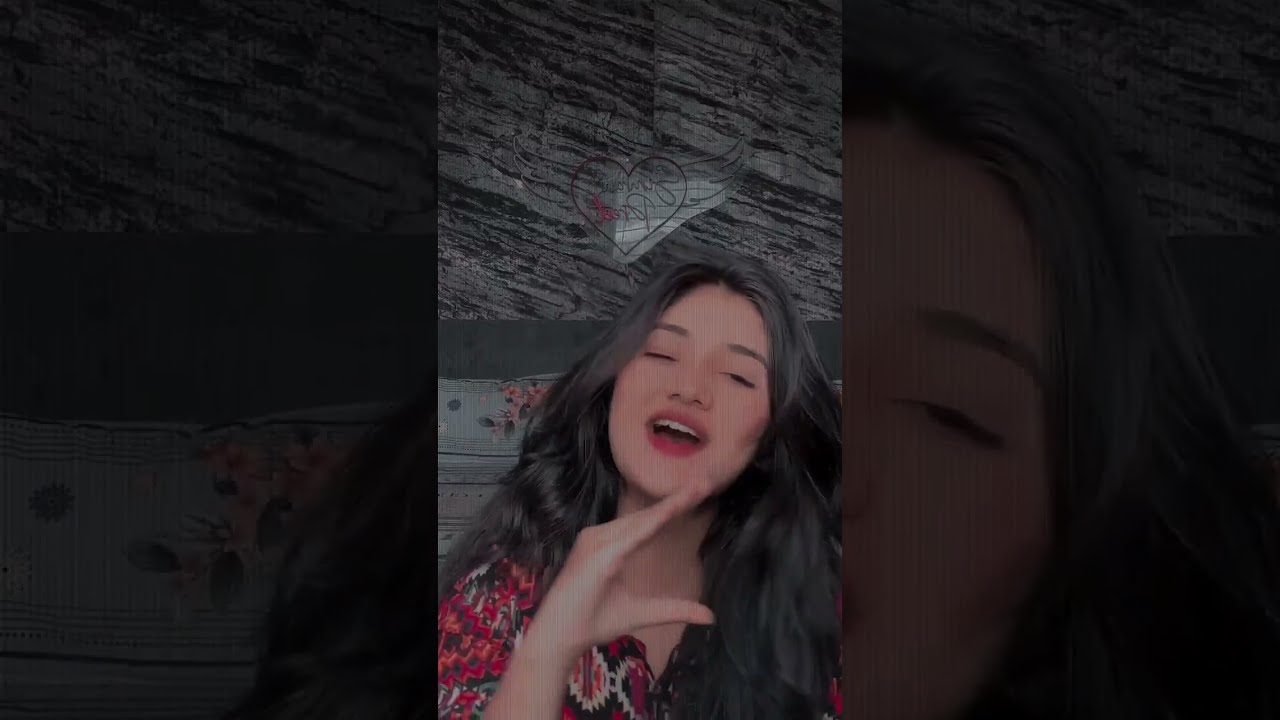The image features a young Asian woman who appears to be in the middle of singing or making a gesture with her right arm forming a shape resembling the letter "C" behind her. She has long, dark black hair and distinct dark eyebrows. Her mouth is open, and her eyes are rolled back slightly, capturing an expressive moment that suggests she might be performing a song. She is wearing a top with an abstract quilted pattern in red, black, and white colors. The background includes a gray and black pattern with a heart and wings motif, and there are pink flowers visible behind her. The overall image has a zoomed-in, slightly blurry or darkened effect, giving it an artistic, album cover-like quality. The setting appears clean, and although there may be some text in the background, it isn't clearly readable.